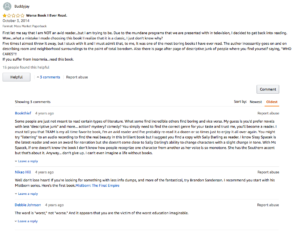The image is a textual document with various colored elements and sections. At the top, there is a small grey circle which appears to have something white inside it, though the details are unclear. Adjacent to this circle is a word. Below this section, there's a yellow element, followed by several lines of text that form a paragraph. Another grey square containing a word appears underneath this paragraph. Following that, there is a sequence of words in different colors: a word in blue, another in grey, and a word or words in black. 

On the next line, the colors alternate between blue and black. Towards the right-hand side, there's a grey rectangle containing a single word, with additional words underneath it. The first two of these words are black, followed by some orange-colored words. 

Further to the right, there's another paragraph, accompanied by words in blue. Another line consists of a mix of words in blue and black, leading to a mostly black paragraph that ends with blue text. The following lines include more blue words interspersed with black. On the right-hand side, several words in black text are present. 

Overall, the document is a mixture of colored text and paragraphs, creating a visually varied layout.